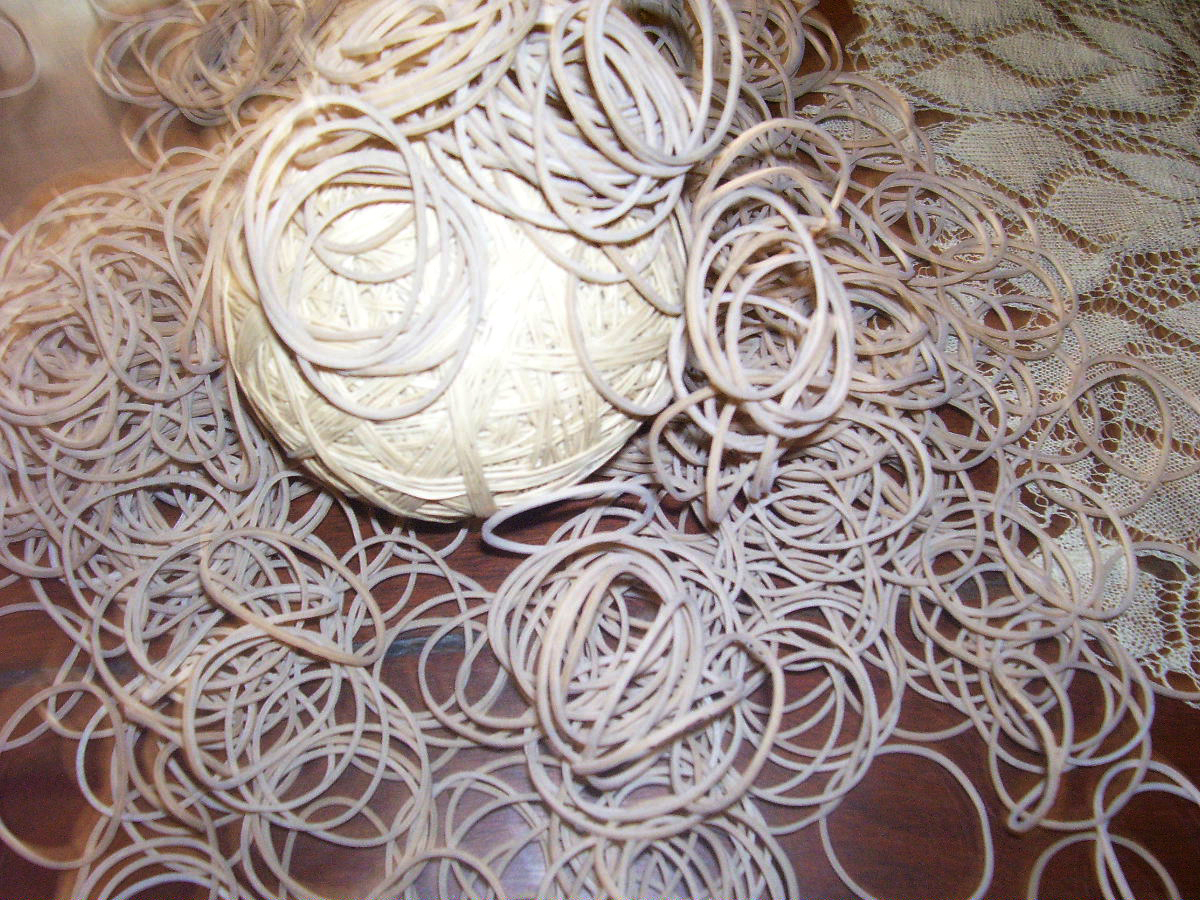An image in landscape orientation shows a dark brown wooden table adorned with a white, lace-like doily. At the center of the scene is a white ball of yarn, brightly illuminated by a light source in the top left corner of the photograph. The ball is enveloped by a plethora of rubber bands, which also spill across the table surface and onto the doily, creating a scattered, messy appearance. The rubber bands, possibly elastics or hair ties, are strewn in abundance around the ball and cover portions of the table, revealing glimpses of the wood beneath them.